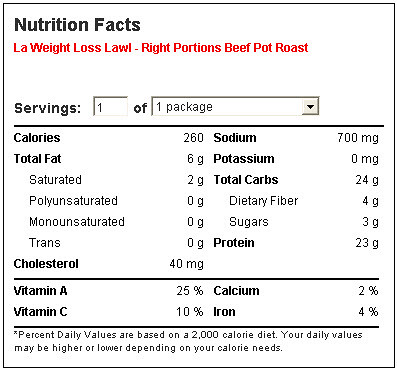The image features a detailed nutritional facts label for L.A. Weight Loss "Right Portions" Beef Pot Roast. The label, predominantly black text with "L.A. Weight Loss" in red, indicates that the single serving package contains 260 calories. Nutritional breakdown includes: total fat at 6 grams, with 2 grams saturated fat, and 0 grams each of polyunsaturated, monounsaturated, and trans fat. Cholesterol content is 40 milligrams, sodium is notably high at 700 milligrams, and potassium is absent at 0 milligrams. Carbohydrates total 24 grams, inclusive of 4 grams dietary fiber and 3 grams sugars. Protein content stands at 23 grams. The label also details percentages of daily values for several vitamins and minerals: 25% Vitamin A, 10% Vitamin C, 2% Calcium, and 4% Iron. It concludes with a standard disclaimer that percent daily values are based on a 2000 calorie diet, with actual daily values varying based on individual calorie needs. The background of the label is not visible in the image.